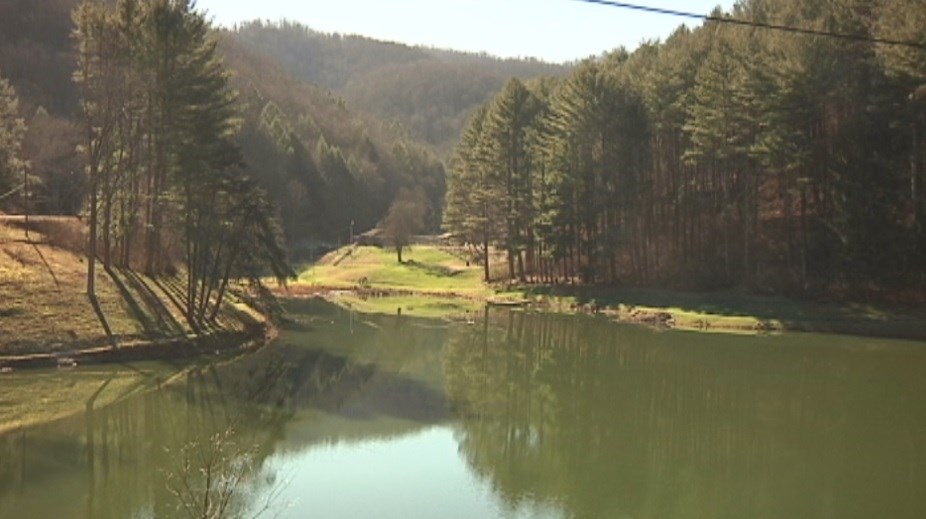The photograph captures a serene mountain lake in landscape orientation, predominantly occupying the bottom part of the image. This calm, light to dark green body of water extends from the foreground towards the horizon and slightly curves to the left, disappearing out of sight. The lake's highly reflective surface mirrors the tall, dark green pine trees that line its grassy, brown-dirt banks on either side. Above, the light blue daytime sky dotted with thin white clouds provides a tranquil backdrop. Surrounding the lake are dense forests and steep hills covered with trees, culminating in a large tree-clad hill in the far distance. The scene, rendered in photographic realism, emphasizes the natural beauty and quietude of the landscape.